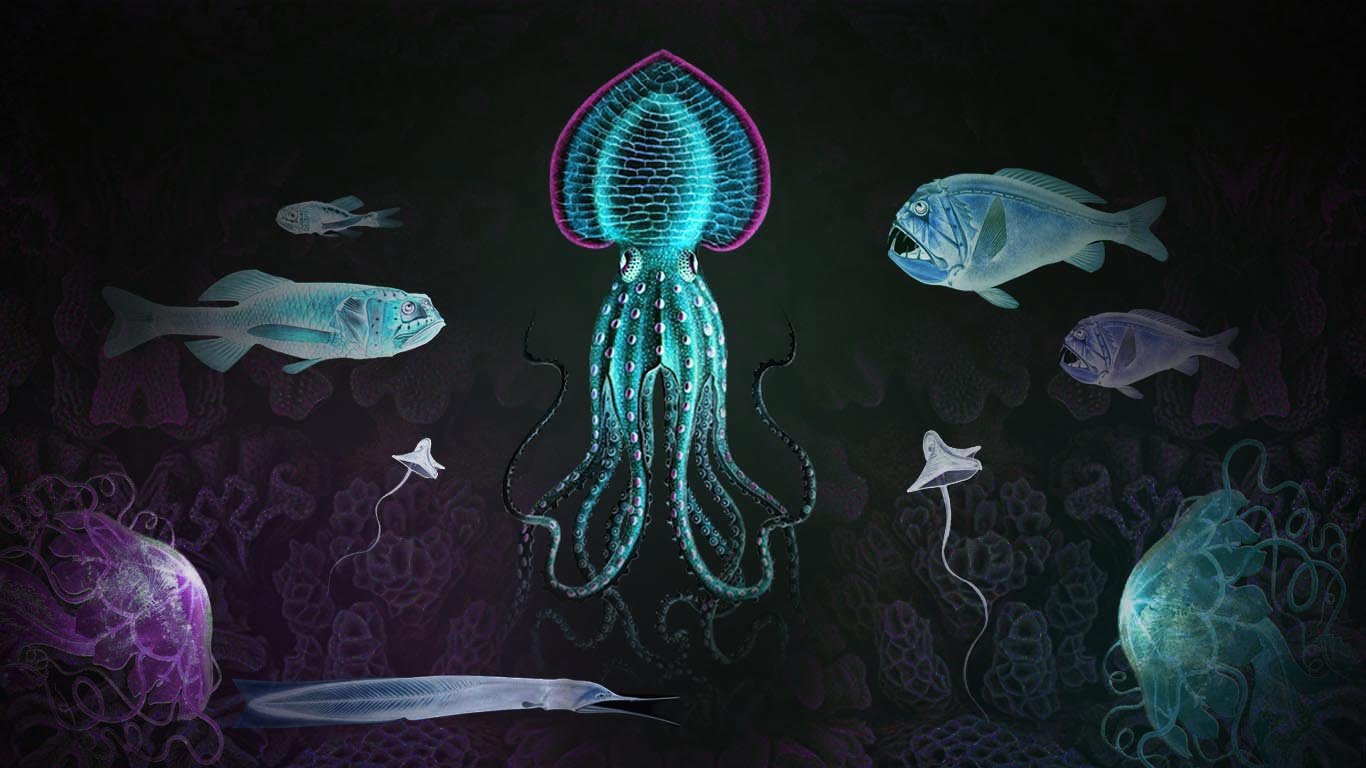In this highly detailed, stylized color illustration, viewers are plunged into a deep-sea underwater scene filled with eerie yet captivating marine life. Dominating the center of the composition is a striking blue octopus with a uniquely spade-shaped head outlined in vibrant magenta. Its body and tentacles are adorned with white spots, creating a mesmerizing pattern that accentuates its surreal beauty. The octopus' eyes are large and white, adding a touch of character to its almost otherworldly appearance. 

Surrounding this central figure are various types of jellyfish that contribute to the image’s haunting allure. Two jellyfish stand out on either side: one on the right is a ghostly turquoise, while its twin on the left is a ghostly purple. Several other jellyfish float ethereally through the scene, some pale and ghostly white, drifting through the murky depths. 

In the foreground, additional deep-sea fish, including some with translucent bodies and long beaks, swim among murky brownish-purple coral formations that resemble morel mushrooms. The background features a shadowy, desaturated expanse, populated by indistinct, spooky blue and purple fish that enhance the eerie ambiance of this underwater ecosystem. The overall composition, with its array of bioluminescent creatures and subtly textured corals set against a mysterious, murky backdrop, evokes a sense of both beauty and eerie tranquility.